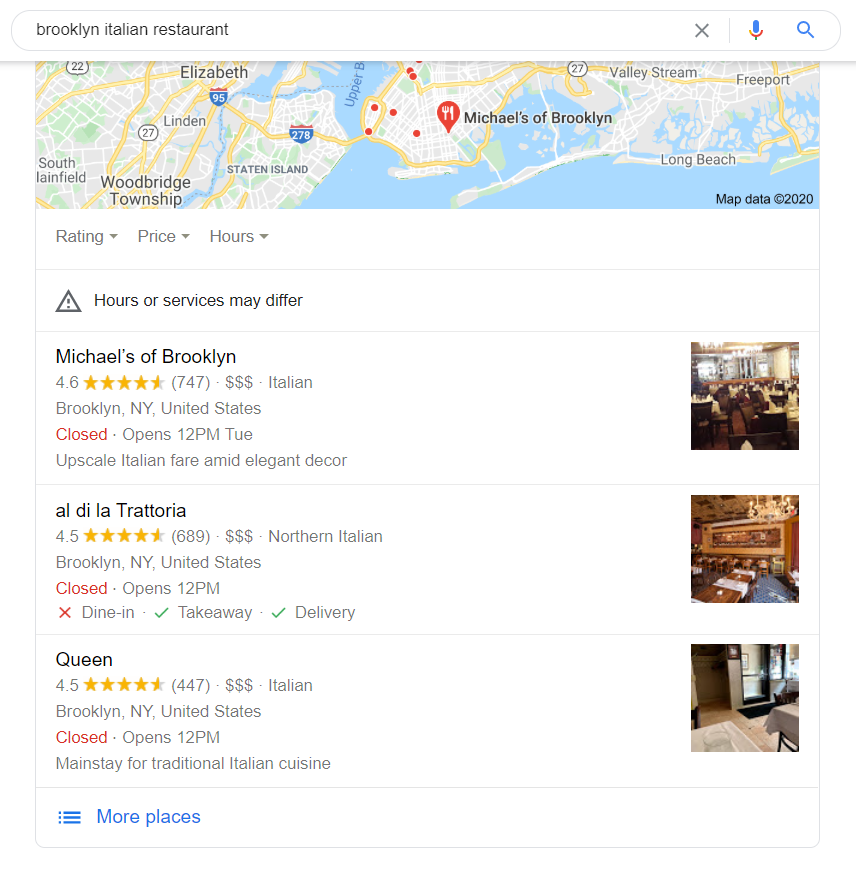The image displays a Google search result for "Brooklyn Italian Restaurant." At the top of the screen is the Google search bar with the search query visible. Below the search bar, a Google Maps snapshot highlights the Brooklyn area in New York City, marked with several red dots and a prominent location pin indicating various Italian restaurants. 

Beneath the map, the first result is "Michael's of Brooklyn," showing a rating of 4.6 stars based on 747 reviews, with a price range indicated by three dollar signs. It is categorized as an upscale Italian restaurant known for its elegant decor. The details reveal that it is located in Brooklyn, NY, United States, and is currently closed, with an opening time of 12 p.m. on Tuesday. 

The second listing is "Al Di La Trattoria," which has a rating of 4.5 stars from 689 reviews and also a price range of three dollar signs, specializing in Northern Italian cuisine. It is located in Brooklyn, NY, United States, and offers dine-in, takeaway, and delivery services. Al Di La Trattoria is also closed at the moment, with a reopening time of 12 p.m.

Lastly, the entry for "Queen" restaurant shows a 4.5-star rating based on 447 reviews, though specific details beyond this point are cut off in the image.

At the bottom of the search results, there is a disclaimer stating, "Hours or services may differ," reminding viewers to check for the most current information.